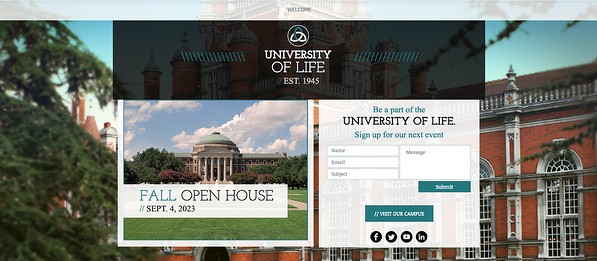**Website Screenshot: University of Life Homepage**

The homepage of the University of Life website features a visually rich background composed of two distinct images divided vertically. On the left side, a striking photograph reveals a lush evergreen tree flanked by green-bricked buildings with various academic steeples and towers adorning the rooftop skyline, evoking the grandeur of a historic campus. On the right, another photograph showcases an architectural masterpiece: a red brick academic building adorned with arched recessed windows set within leaded glass encasements, separated by ornate pillars.

A central pop-up overlays this scenic backdrop. At the very top center, a black bar prominently displays the university's name, "University of Life," in white font, along with the establishment year, 1945. Above this text, a circular logo featuring intertwining white and green leaves adds a touch of elegance.

To the left within the pop-up, a photograph of an ivory-colored, multi-story stone building with a central rotunda and a front colonnade is prominently featured. Overlaying this image, a white bar announces the "Fall Open House, September 4, 2023."

On the right side of the pop-up, there's a clean and inviting form titled "Be a part of the University of Life. Sign up for our next event," with "University of Life" in black text and the rest in green. The form includes input fields for name, email, subject, and message, all in white boxes. Beneath these fields, a green pill-shaped button enables users to submit their information. At the very bottom, another green bar, clickable, is labeled "Visit Our Campus" with a hashtag symbol at the front.

Underneath this form are four black social media icons, each housed in a black circle: a Facebook "F," a Twitter bird, and an "IN" for LinkedIn, encouraging visitors to connect and engage on social platforms.